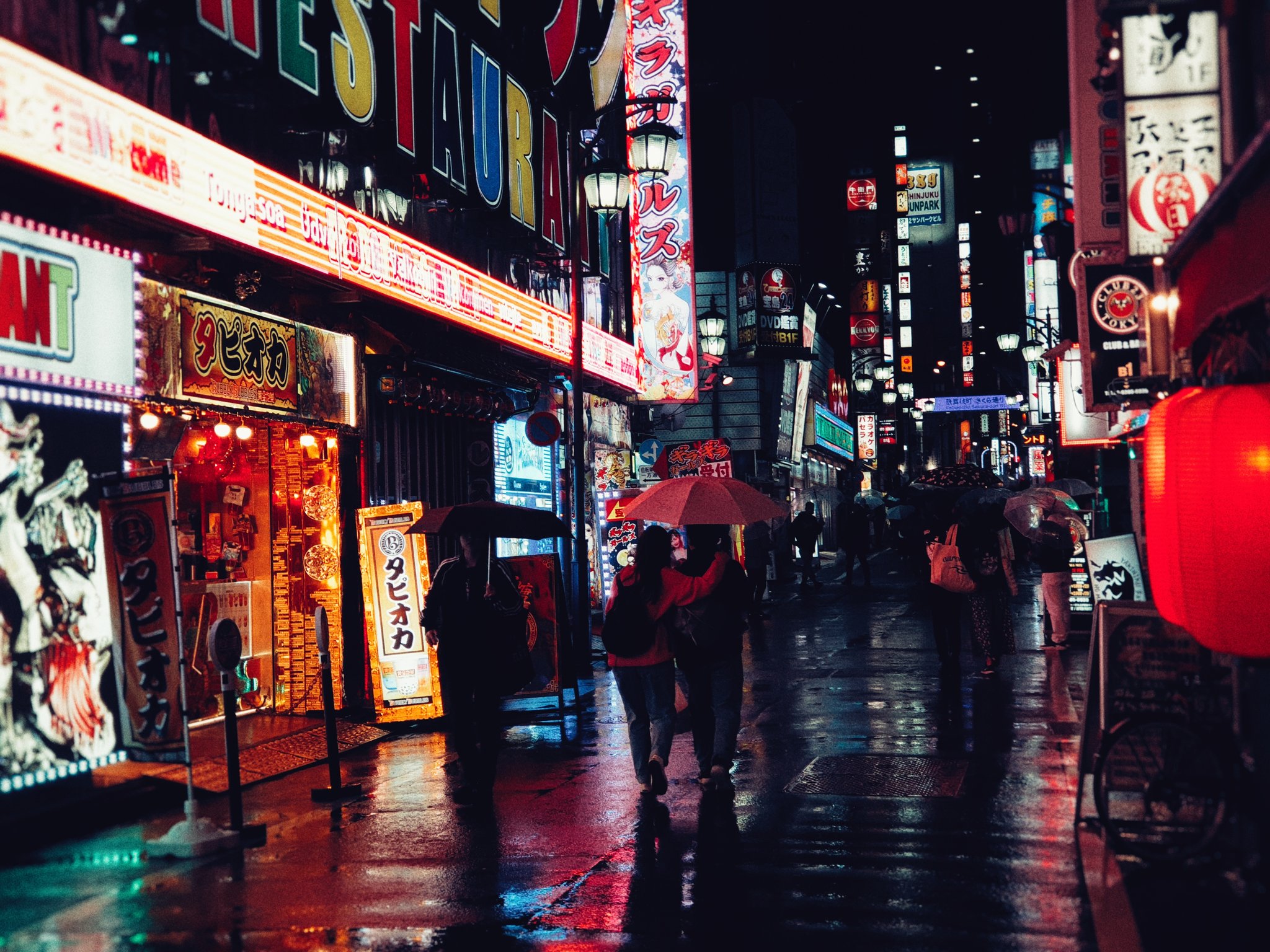This is a captivating color photograph depicting a bustling city street at night, likely in Japan, as suggested by the "Club Tokyo" sign and prevalent Asian script on the signage. The street, adorned with an array of neon signs and marquees in vivid hues of red, purple, orange, yellow, and white, is illuminated by a mix of these colorful lights and the glow from a red Chinese lantern on the right. The rain-slicked pavement has prompted pedestrians to wield umbrellas, adding to the scene's dynamic feel; notably, there's a striking red umbrella among the several black ones. The people, clad in various attire including a red sweater and all-black outfits, walk away from the viewer, their backs to the camera. An orange storefront is visible on the left, while numerous signs, some partially obscured but including the English word "restaurant," contribute to the dense, vibrant ambiance of this pedestrian-only street, devoid of cars. The encompassing buildings recede into the distance, all bathed in the colorful glow of the urban landscape under a pitch-black sky.